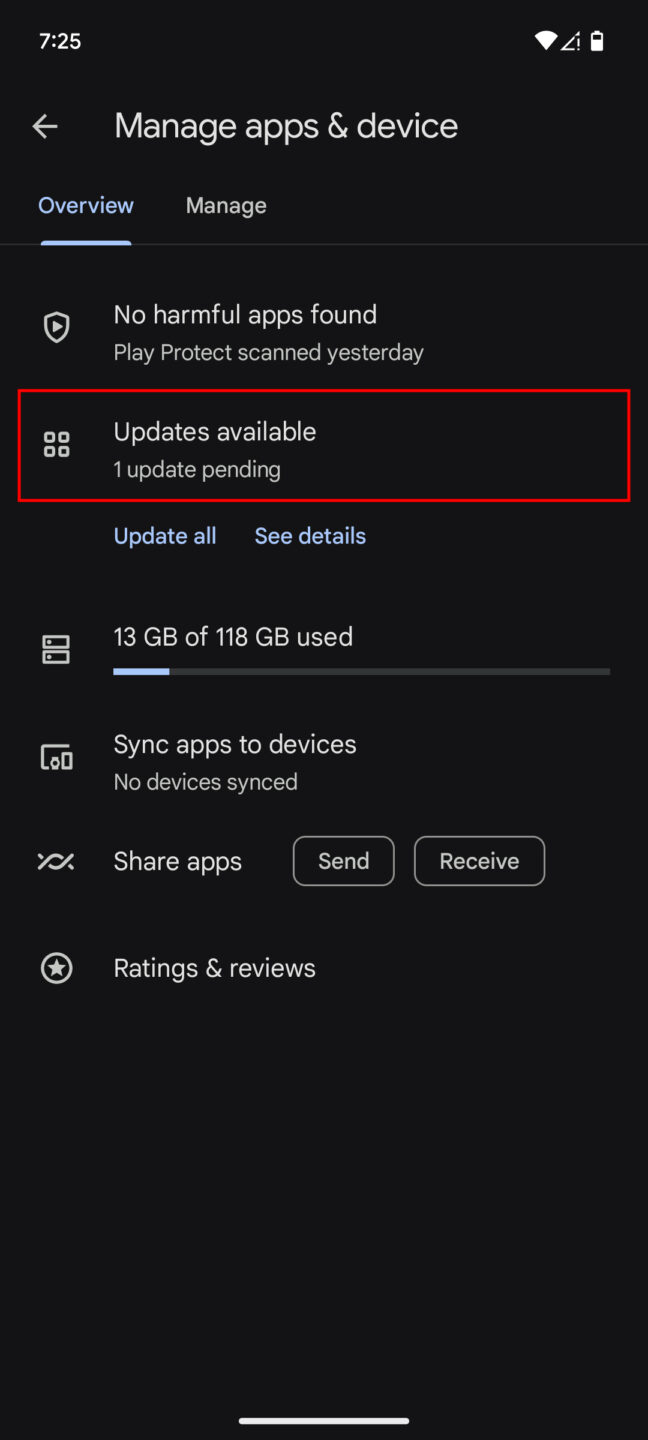The image depicts a close-up view of a cell phone screen showcasing various system information and settings. The screen indicates the current status, including 4 out of 5 signal bars, active Wi-Fi, and a battery charge at approximately 75%. 

At the top, the screen displays the heading "Manage apps and devices" with a left arrow icon. Below this are two tabs: "Overview" and "Manage." The "Overview" tab is highlighted in blue with a blue underline, signifying it as the active selection. 

The displayed "Overview" screen includes several pieces of information:
- **No harmful apps found**: Play Protect scan completed yesterday. 
- **Updates available**: Highlighted with a red rectangle, indicating one update is pending with an option to "Update all" or "See details" in blue text.
  
Further down, it shows storage usage: **13 GB used out of 118 GB**. A blue progress bar indicates minimal storage usage.

Additional sections include:
- **Sync apps to devices**: Status shows no devices are synced.
- **Share apps**: Options to "Send" or "Receive."
- **Ratings and Reviews**: Section primarily in white text.

The user interface features a black background with predominantly white text, accented by blue text and highlights, and is punctuated by a red rectangle around the updates section. A white bar is positioned at the very bottom center of the screen.

This detailed summary highlights the structured and diverse details visible on the cell phone screen.